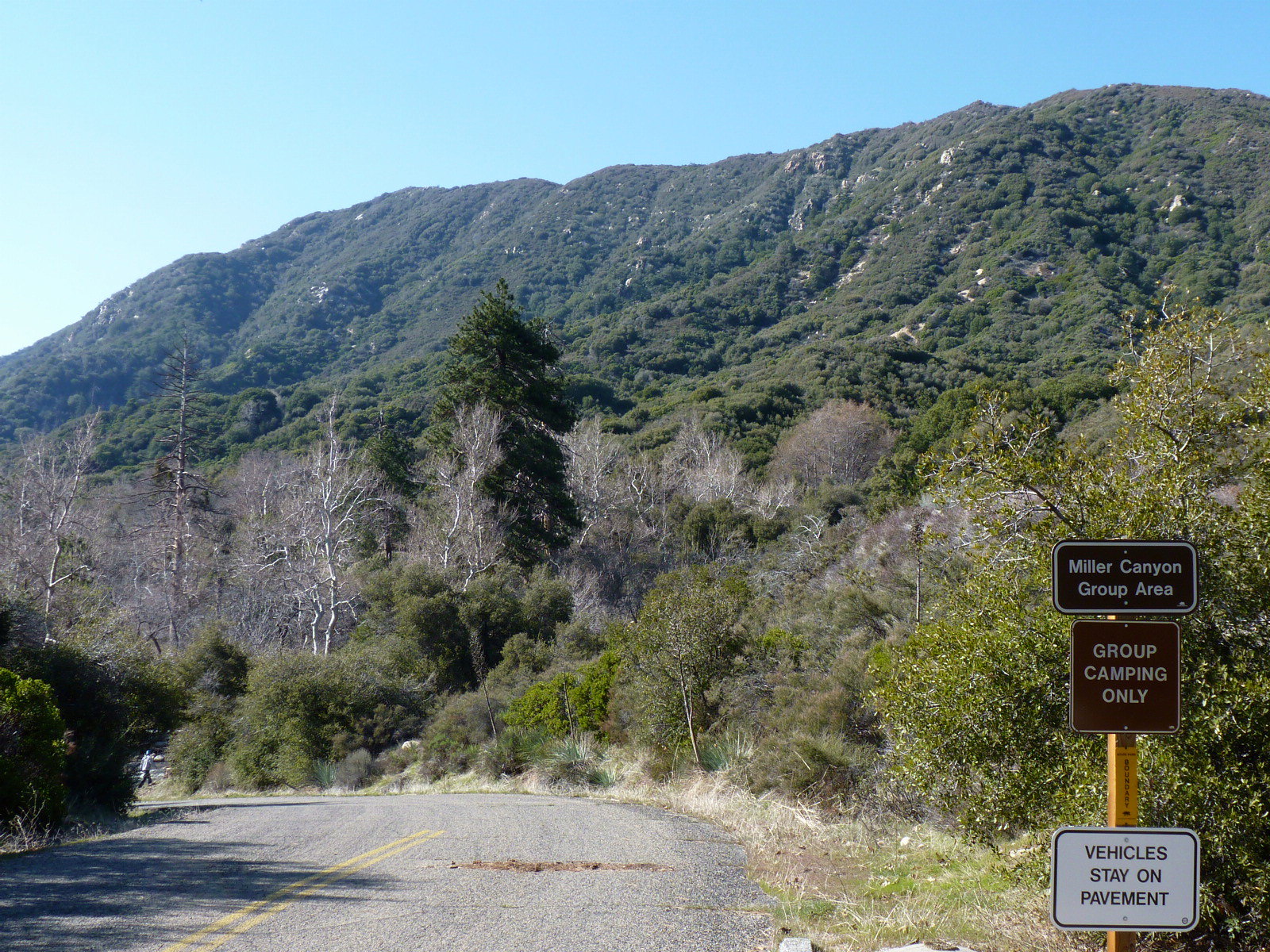The image captures a scenic view of Miller Canyon Group Area, an outdoor camping site nestled within a mountain range. Dominating the background is a vast, imposing mountain adorned with varying shades of green, gray, and brown trees, some in full bloom while others stand barren with light brown branches. The sky above is a light blue, providing a serene contrast to the dense foliage below. In the foreground, a curved, two-lane asphalt road with a double yellow line winds from the bottom left corner, flanked by bushes and additional trees. On the far right of the image, a series of signs on a single post direct campers: a brown sign reads "Miller Canyon Group Area" above another stipulating "Group Camping Only," and the lowest sign on a white background instructs "Vehicles Stay on Pavement." The scene, likely captured casually by a visitor, is rich in natural hues and combined details, highlighting the rustic tranquility of this mountainous canyon camping area.